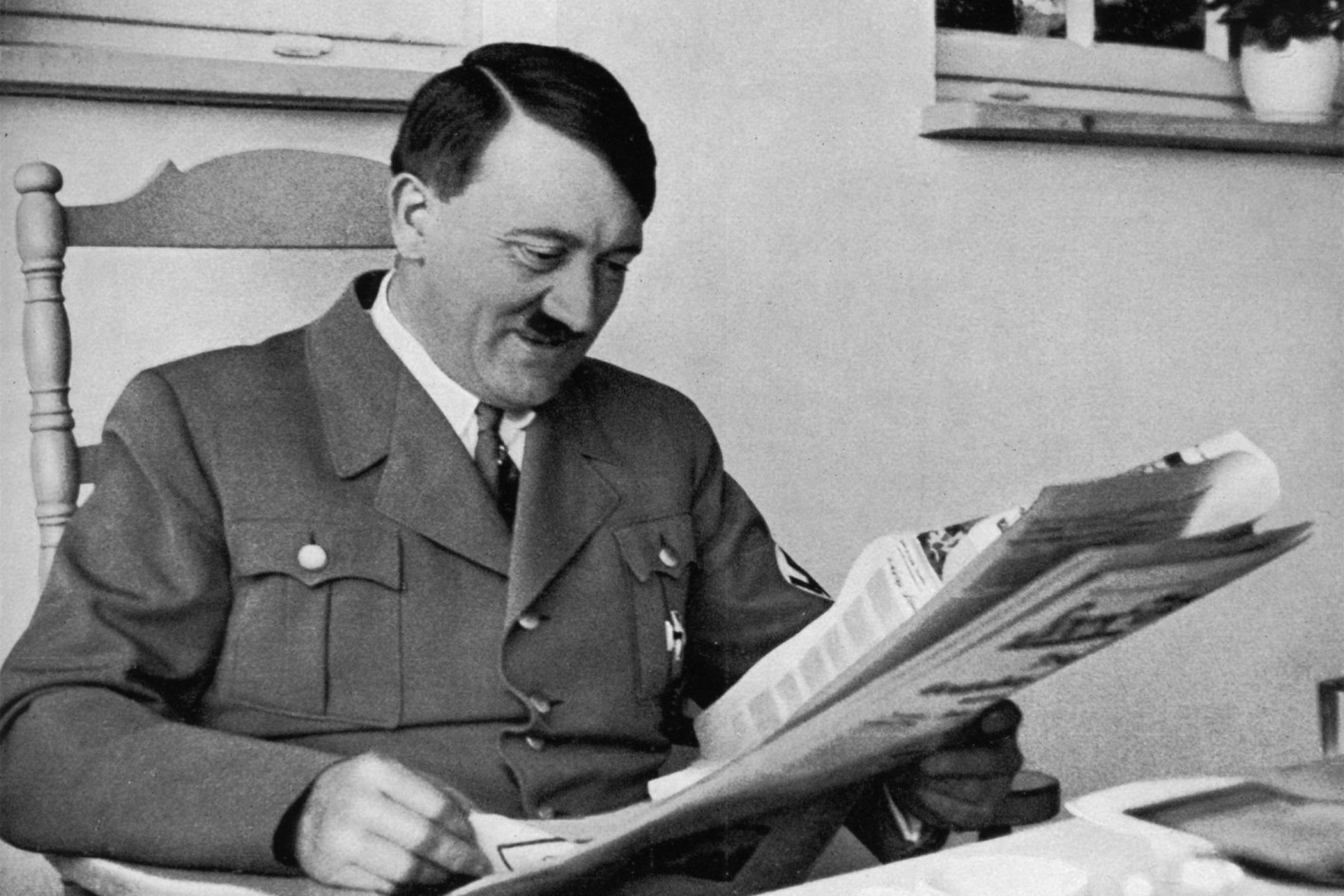This black and white photograph captures Adolf Hitler seated in an old-fashioned wooden chair. The image cuts off at his midsection, showing him dressed in his German Army outfit jacket, with a white button-down shirt and a tie underneath. Hitler's brown hair is neatly parted on the side, and he wears his characteristic mustache. He is smiling with his mouth closed as he looks down at a newspaper he holds in both hands. The setting appears to be indoors, possibly a dining or kitchen area, suggested by a table with a white tablecloth and a cup in the lower right-hand corner. Behind him is a plain white wall with the bottoms of two windows visible, one of which has a potted plant on the windowsill.